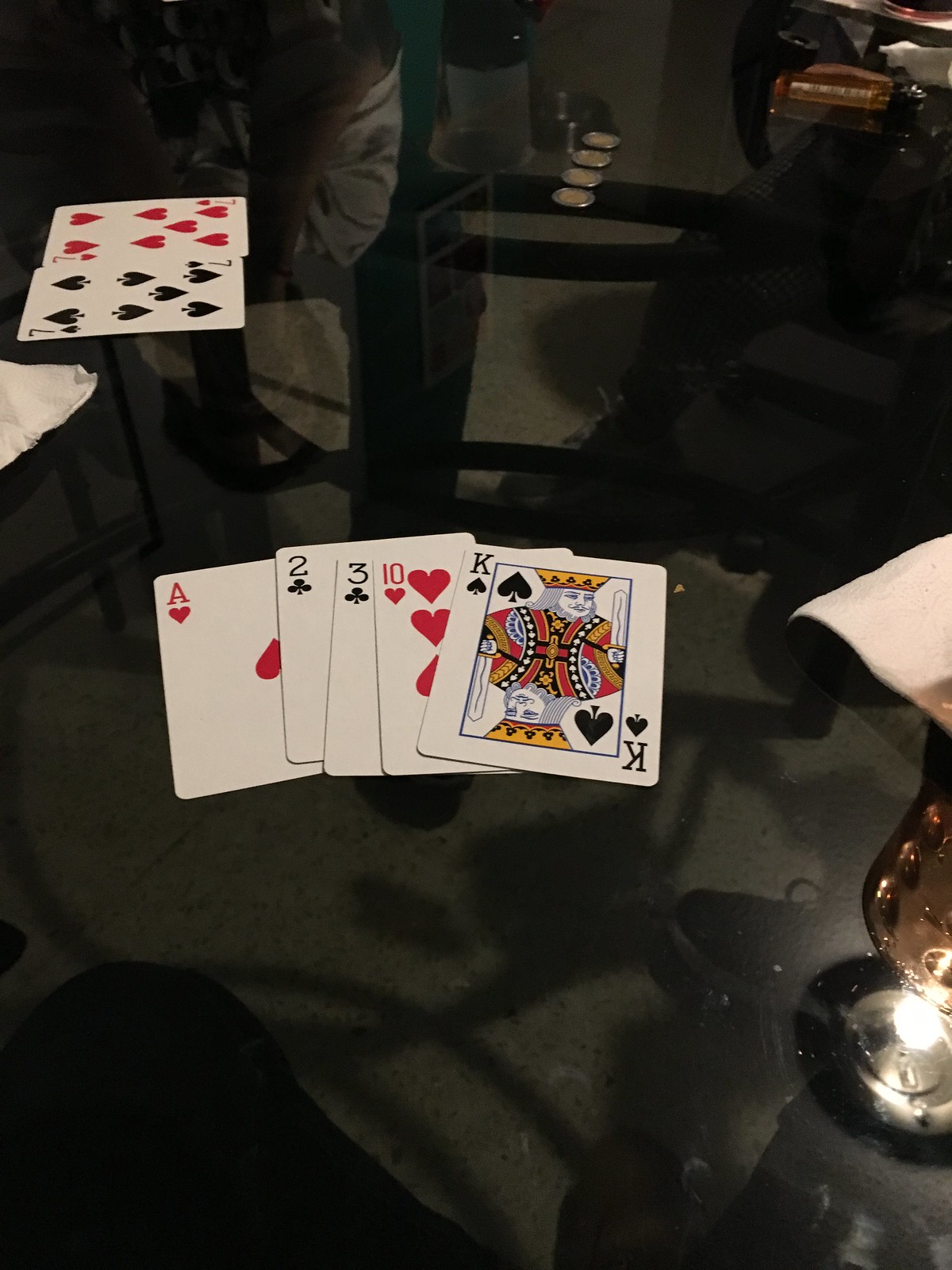The image depicts seven playing cards sprawled across a table covered with a dark tablecloth. Arranged in a seemingly random fashion, two cards are positioned in the background: the Seven of Hearts and the Seven of Spades. Dominating the foreground, five cards lie in closer view, comprising the Ace of Hearts, the Two of Clubs, the Three of Clubs, the Ten of Hearts, and the King of Spades. Resting beside the cards is a mysterious golden object topped with a light pink accent, potentially a candlestick, adding a touch of intrigue to the scene. The vibrant red and stark black suits contrast sharply against the otherwise muted background, with the cards themselves placed on a standard white surface typical of playing cards. No writing or additional elements clutter the image, lending it an air of simplicity and focus on the cards.